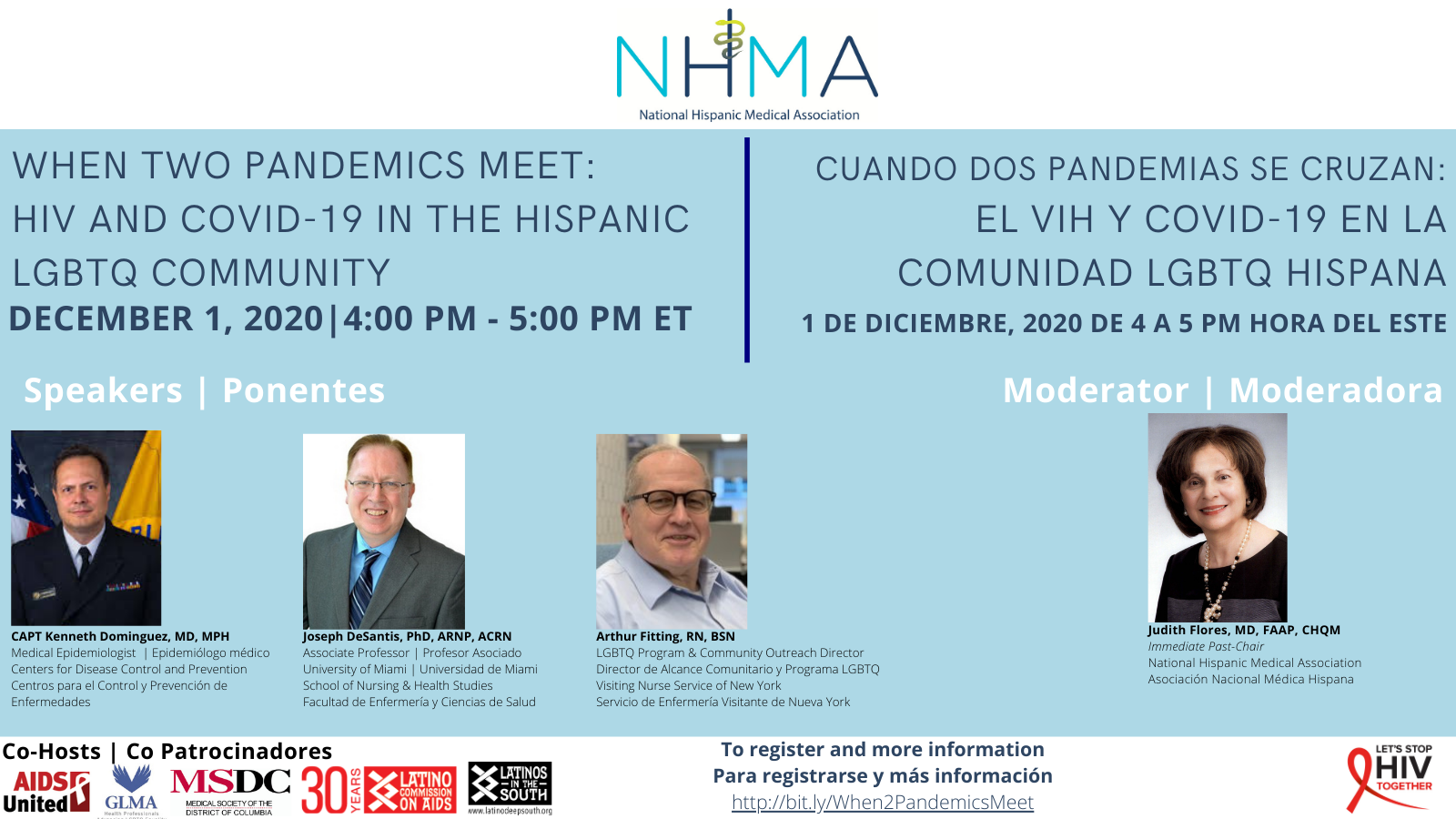This is a landscape-oriented flyer with a light blue background promoting an event organized by the National Hispanic Medical Association (NHMA). At the top, in a combination of light and dark blue text, it reads "NHMA National Hispanic Medical Association". Below that, bold text announces the event: "When Two Pandemics Meet: HIV and COVID-19 in the Hispanic LGBTQ Community," scheduled for December 1st, 2020, from 4 to 5 p.m. Eastern. 

The left side of the flyer features headshots of three speakers: Captain Kenneth Dominguez, Joseph DeSantis, and Arthur Fitting, with their names and titles displayed prominently underneath. 

On the right side, the same event details are provided in Spanish: "Cuando dos pandemias se cruzan: VIH y COVID-19 en la comunidad LGBTQ Hispana," along with the same date and time. This side also features a headshot of the moderator, Judith Flores, identified as the immediate past chair and moderator for the event.

At the bottom of the flyer are colorful logos of various organizations co-hosting the event, including AIDS United, GL, MSDC, the Latino Commission on AIDS celebrating 30 years, and Latinos in the South.